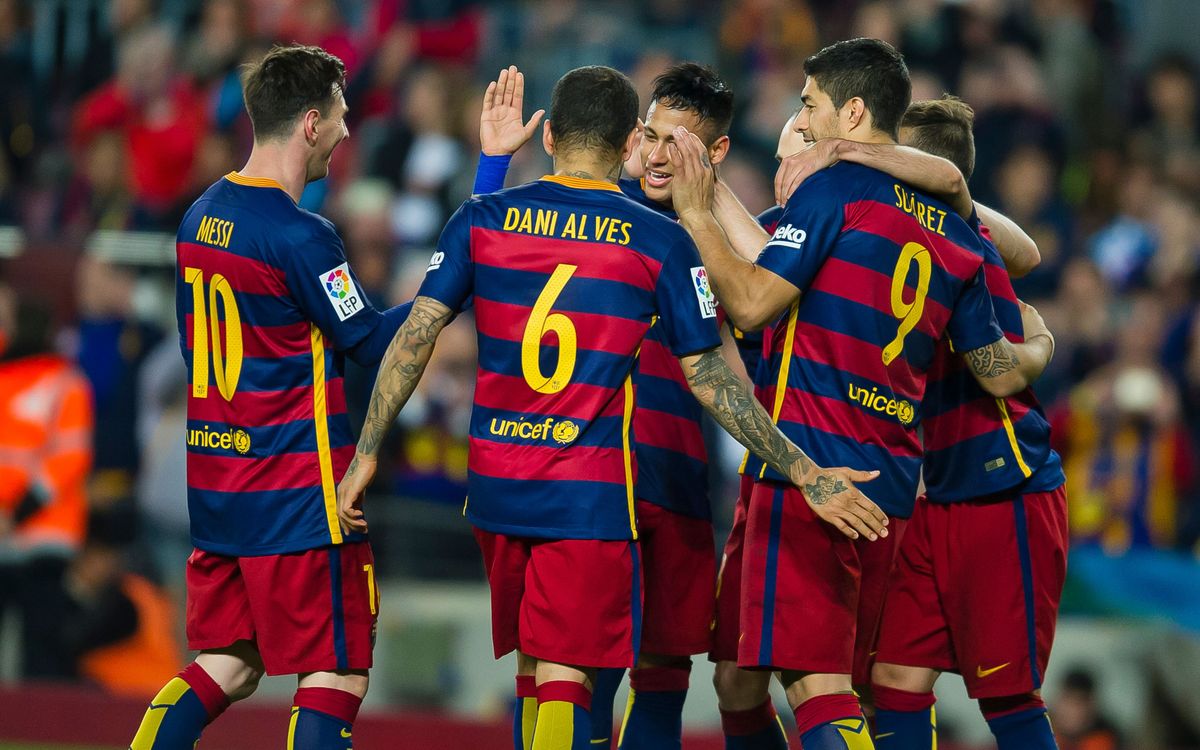This photo captures a celebratory moment featuring Barcelona players, prominently showcasing Dani Alves, Lionel Messi, and Luis Suarez. They are standing close together in the middle of the field, smiling, giving high-fives, and embracing each other, clearly reveling in their victory. Messi is identifiable by his number 10 jersey, Dani Alves by his number 6, and Suarez by his number 9. The players are dressed in Barcelona's iconic blue and red striped uniforms with matching shorts. While the background is blurred, it’s evident that a large crowd of spectators is watching from the bleachers, further emphasizing the team's focal point in this moment of triumph.